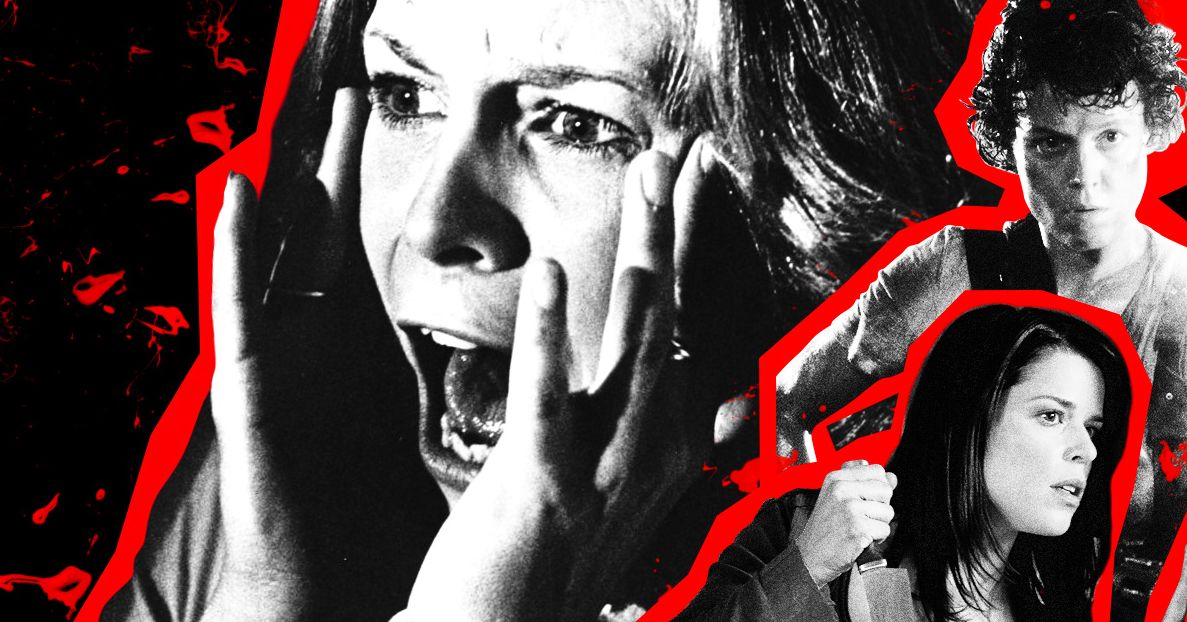This mixed-media collage presents a harrowing montage of three figures set against a stark black background. Dominating the composition is a large, black-and-white portrait of a woman, her hands clasping her face in a scream of palpable terror. This central figure is flanked by a pair of equally unsettling images—a person, likely Sigourney Weaver, appearing in the upper right, and another woman, possibly Neve Campbell, in the lower right, both displaying expressions of fear. The woman in the lower right has shoulder-length hair that curls inward at the ends and holds her hand in a tense fist. Vibrant red lines and splashes act as borders around each individual, adding a sharp contrast and tying the figures together. The red touches also form abstract shapes in the background, resembling keys or other ambiguous forms, enhancing the eerie and fragmented nature of the artwork.